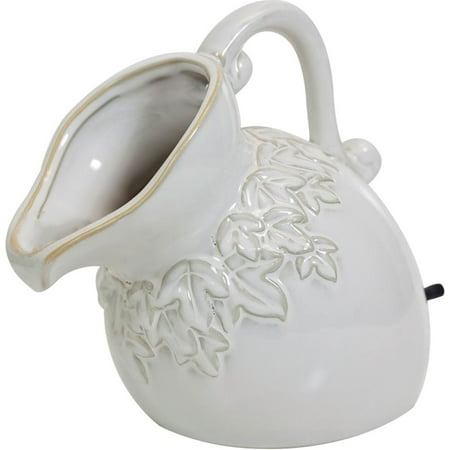This image is a stock photograph of an off-white ceramic pitcher set against a plain white background. The pitcher features a bulbous, slightly off-center base, giving it a unique, handmade appearance. Its wide mouth and spout are accented with a mustard-colored piping around the lip, adding a subtle touch of color. The pitcher is decorated with embossed grape leaves that encircle its neck, with gray outlines where the paint hasn't fully covered the relief pattern. The handle at the back is round and adorned with curlicues on both ends, imparting an elegant touch. Additionally, there is a small black tab on the right-hand side, although its function is unclear. The pitcher, with its artistic design and organic shape, exudes a rustic charm.